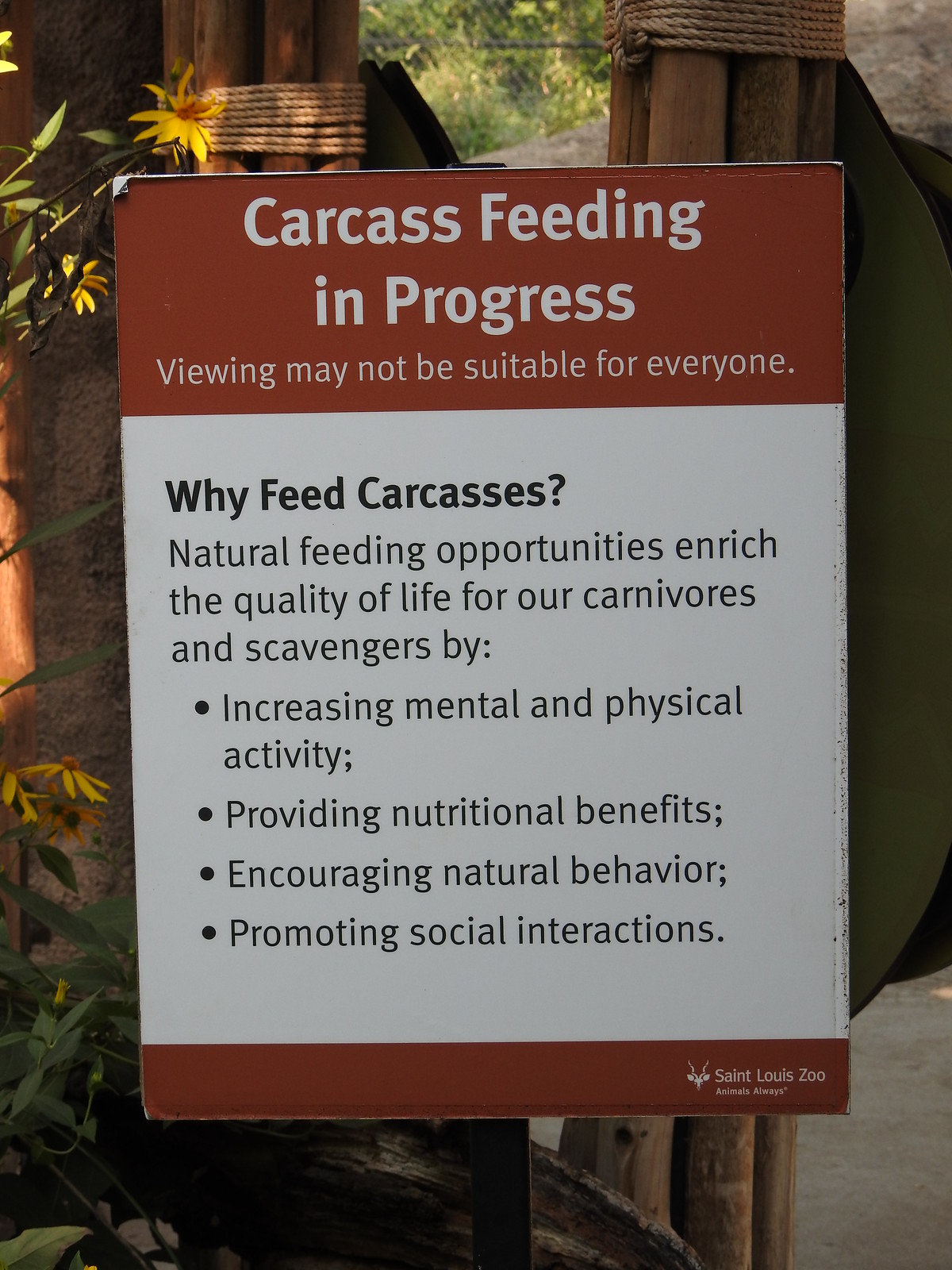This detailed image captures an informative outdoor sign at a zoo, framed by a naturalistic and structured backdrop. The sign itself is rectangular, tall, and predominantly white, bordered by a large burnt red rectangle at the top and a slightly smaller one at the bottom. The crisp white font on the top red border states, "Carcass feeding in progress. Viewing may not be suitable for everyone."

Beneath this warning, the white background of the sign elaborates, "Why feed carcasses? Natural feeding opportunities enrich the quality of life for our carnivores and scavengers by increasing mental and physical activity, providing nutritional benefits, encouraging natural behaviors, and promoting social interactions."

The setting around the sign enhances its context: you can see several yellow flowers and green tree foliage, accented by a gate in the background. Prominent behind the sign are two tall wooden poles, composed of several smaller poles tightly bound together with light brown rope, indicating a rustic, well-integrated zoo environment. On the left side, there appears to be the trunk of a tree, adding to the natural ambiance of the scene. This thoughtful setup suggests the sign is informing visitors about the potentially unsettling but natural feeding practices necessary for the well-being of carnivores and scavengers, possibly including tigers or other meat-eating animals.